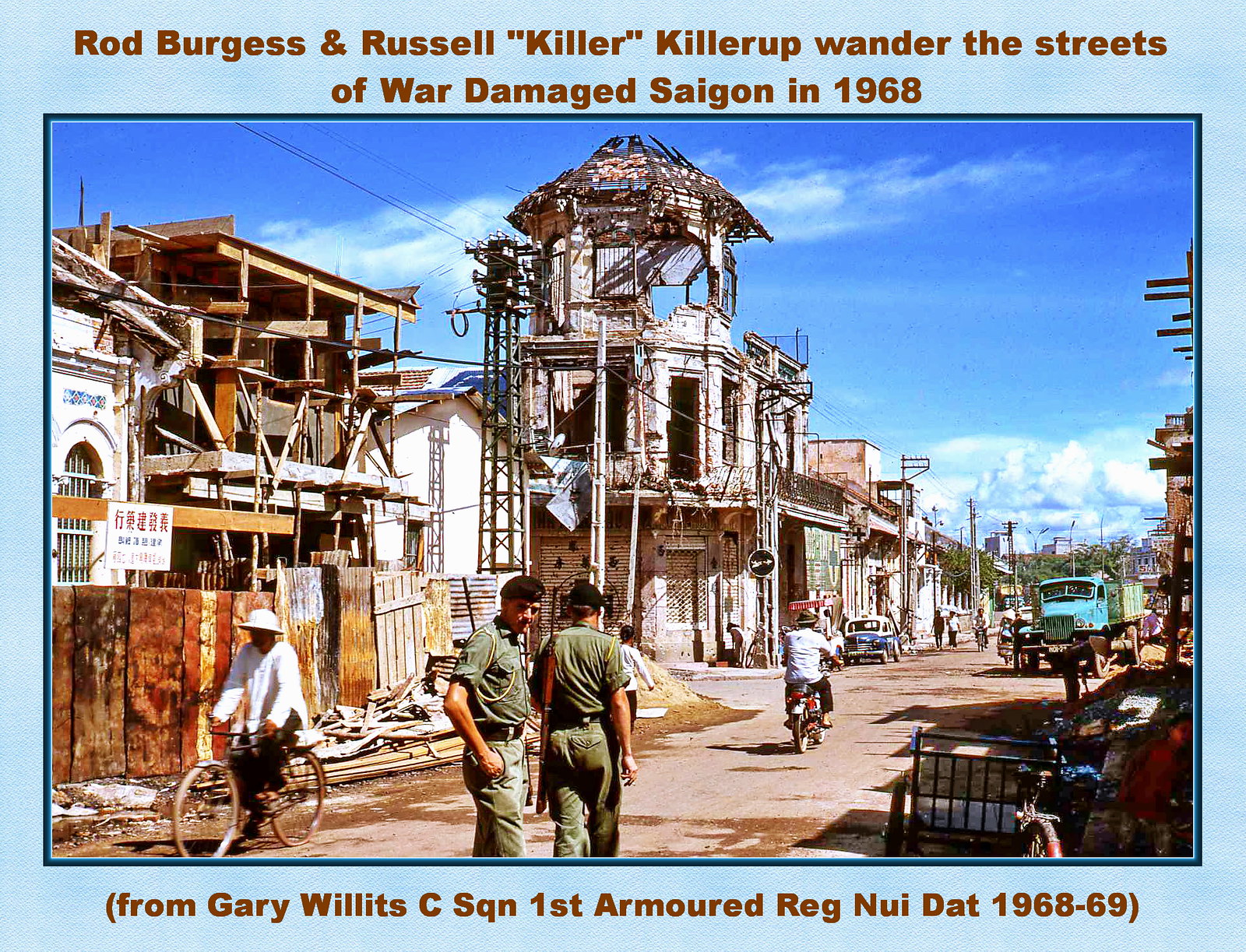In this war photograph titled "Rod Burgess and Russell Killarup Wander the Streets of War-Damaged Saigon in 1968," we see a clear portrayal of the ravages of war. Two soldiers, dressed in green uniforms and berets, walk the dirt streets, their rifles in hand. One soldier looks directly into the camera with his hands in his pockets, while the other, with his back to the camera, rests his gun on his left shoulder. These streets are lined with heavily damaged buildings, some retaining only the remnants of their façades, now mere ruins and relics of their former structures. The daytime sky is blue and clear, with white clouds contrasting the scene below. Among the debris, Vietnamese people in traditional attire, complete with hats, bicycle around the streets, indicative of their attempts to continue daily life amidst the chaos. In the background, a truck and a 1950s taxi can be seen, parked alongside the road. Most people in the scene navigate these war-torn streets on bicycles. The photograph also bears a footnote at the bottom that reads, "From Gary Wilkes, C-Squadron, 1st Armored Regiment, Nui Dat, 1968-69".